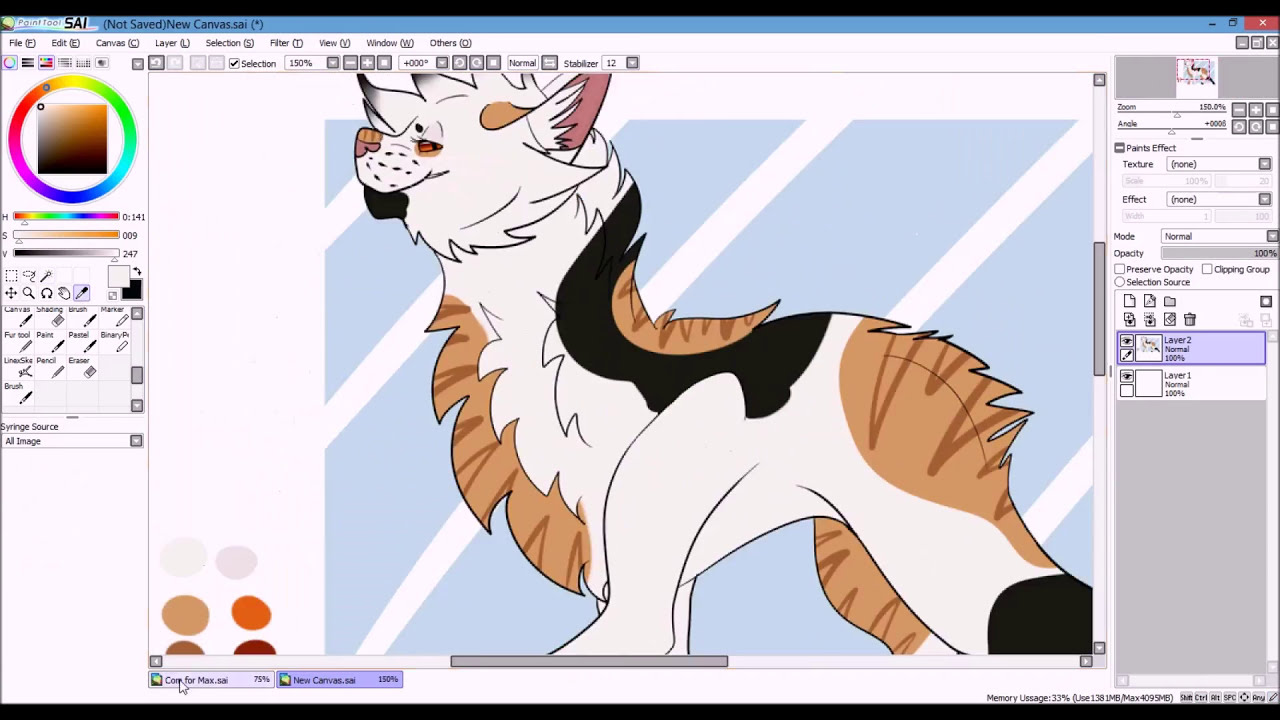The image depicts a computer screen displaying a digital art program. The screen is framed by thin black rectangles at the top and bottom. At the very top, there is a blue gradient strip with an X on a red box at the right end. On the left side of the screen, against a white background, there is a color wheel and several white square icons featuring paintbrushes. The right side of the screen showcases a gray and white menu bar with different options like texture, effect, and mode. Central to the display is a drawing space with a blue and white striped background. The artwork itself appears to be a stylized side portrait of an animal, resembling a cross between a tiger and a wolf. It has striking features including large white ears with pink interiors, red eyes, and an expressive smile. Its fur is predominantly white with patches of black and light brown. Notably, the fur around its chest, back, and part of the tail is brown, while the rest of its body is white, creating a pattern of intricate details. The creature is facing left, showcasing its long legs and bushy, light brown-streaked fur, accented by small triangle patterns.